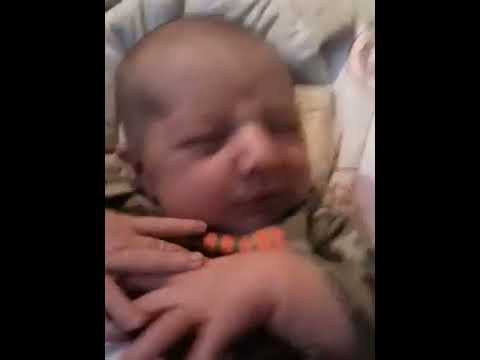This slightly blurred photograph captures a very young baby, possibly just a few weeks old, with fair, peach-toned skin and sparse hair. The baby, eyes closed and hands resting clasped on its chest, is dressed in a dark green shirt adorned with some indistinct orange lettering near the neck. Positioned in what appears to be a rocker or bassinet, the baby is nestled against a light blue cushioned backdrop. The image is framed by two vertical black strips on either side, adding a sense of enclosure around the peaceful scene. Scattered colors in the background, including cream, white, and pink, hint at additional bedding or soft furnishings, contributing to the cozy and tender atmosphere.